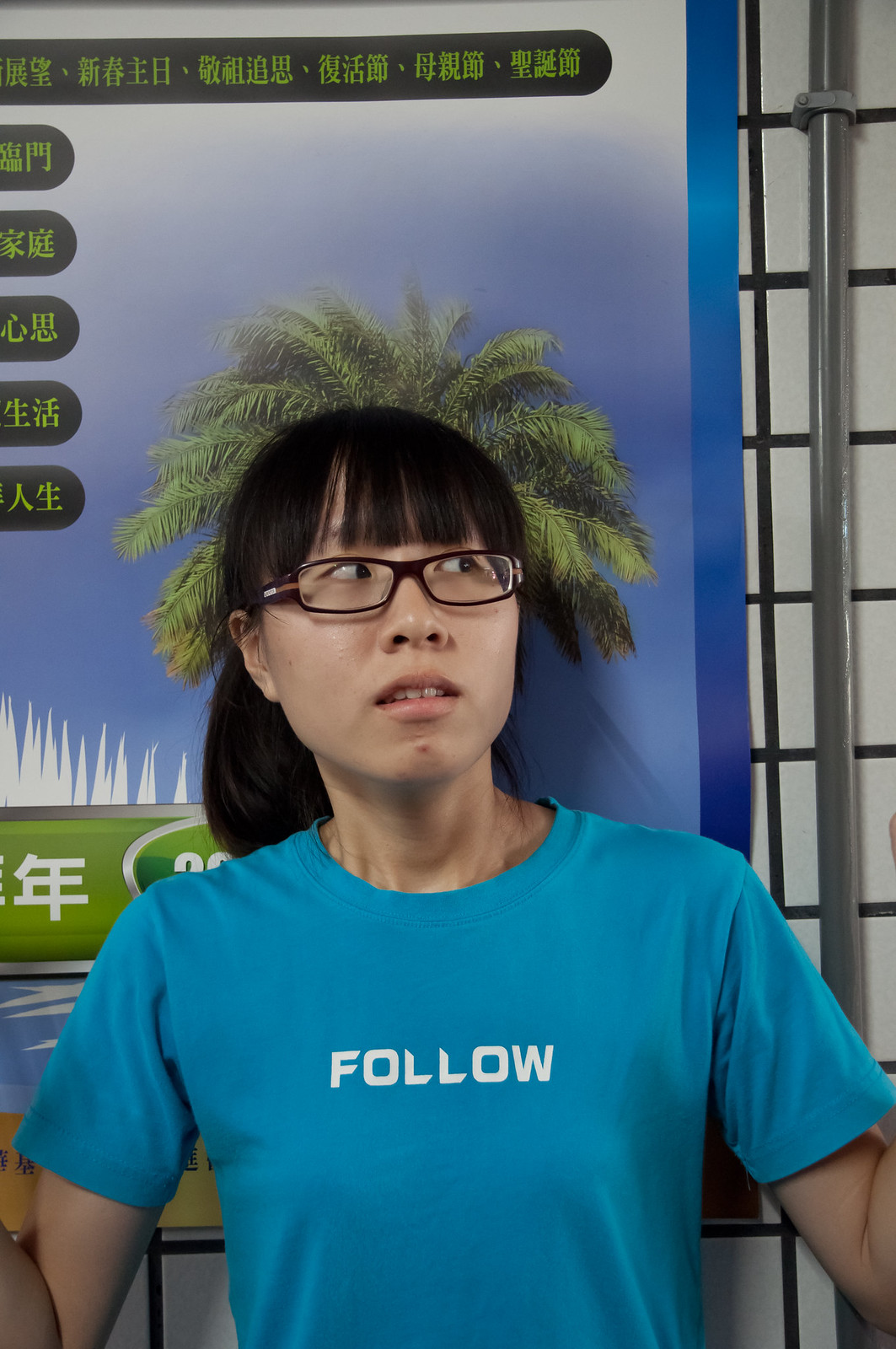This image portrays an Asian woman standing against a wall with white square tiles featuring black grout lines. She has long black hair with bangs that fall below her eyebrows, and she's wearing rectangular brown-framed glasses. Her expression is curious or apprehensive, with her eyes directed to the left and her mouth slightly open.

The woman is dressed in a blue T-shirt with the word "FOLLOW" prominently written in white capital letters in a distinctive font. Behind her is a blue poster board bordered in the same color, which features a large green palm tree. The leaves of the palm tree are positioned such that they humorously appear to sprout from her head, giving the illusion of green, frizzy hair. Additionally, there are black labels with green text on the poster, which likely include neon green-colored Asian characters. 

A visible silver conduit pipe runs along the tiled wall, adding an industrial element to the scene. This intricate setup, combined with the woman's expressive look and the playful positioning of the palm tree, makes for an engaging and slightly comical photograph.